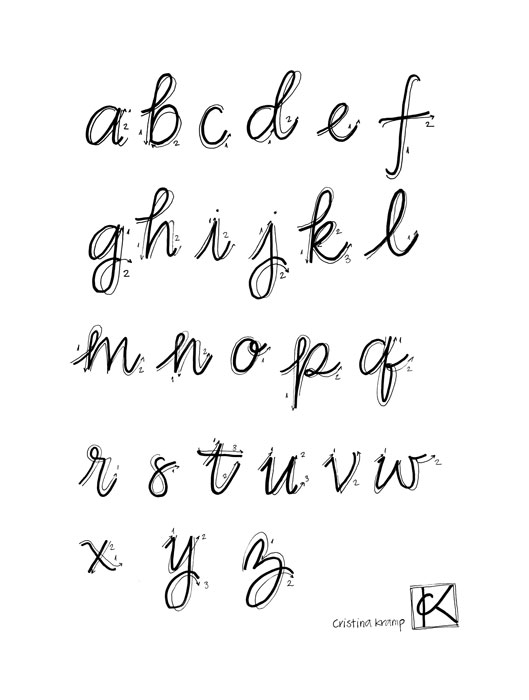The image features the entire cursive alphabet from A to Z written in black ink against a white background. The cursive letters are arranged in five rows, with the first four rows containing six letters each and the final row containing three letters. Small numbers, ranging from 1 to 4, are positioned around each letter, likely as a guide for how to write them. In the bottom right corner, the name "Christina Kramp" is inscribed alongside a custom black and white logo, which features the initials "CK". The text appears to be created with a handwritten font, offering a sleek and personalized touch.